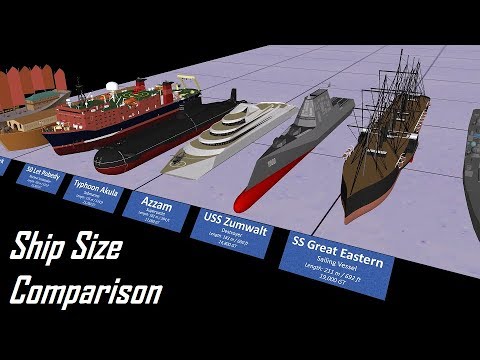The image is a computer-generated illustration designed to compare the sizes of various ships. It features a black background with a white surface at the bottom, on which the ships are displayed in a row from right to left. Each ship is labeled with blue placards featuring white text. The larger ships appear on the right side, while smaller ones are positioned to the left, becoming harder to read as they recede into the distance. The prominent white text in the lower left-hand corner reads "Ship Size Comparison."

Starting from the right, the ships are labeled as follows: the first ship, a large sailing ship, is identified as SS Great Eastern. The next ship, a gray and red destroyer, is labeled USS Zumwalt. Following that is a white luxury yacht named Azzam. Next is a submarine called Typhoon Akula, colored black. To the left of that is a vessel labeled Let Peabody, and there’s another ship further left whose label is unreadable. The image provides an informative comparison showcasing the varying sizes of these notable ships.